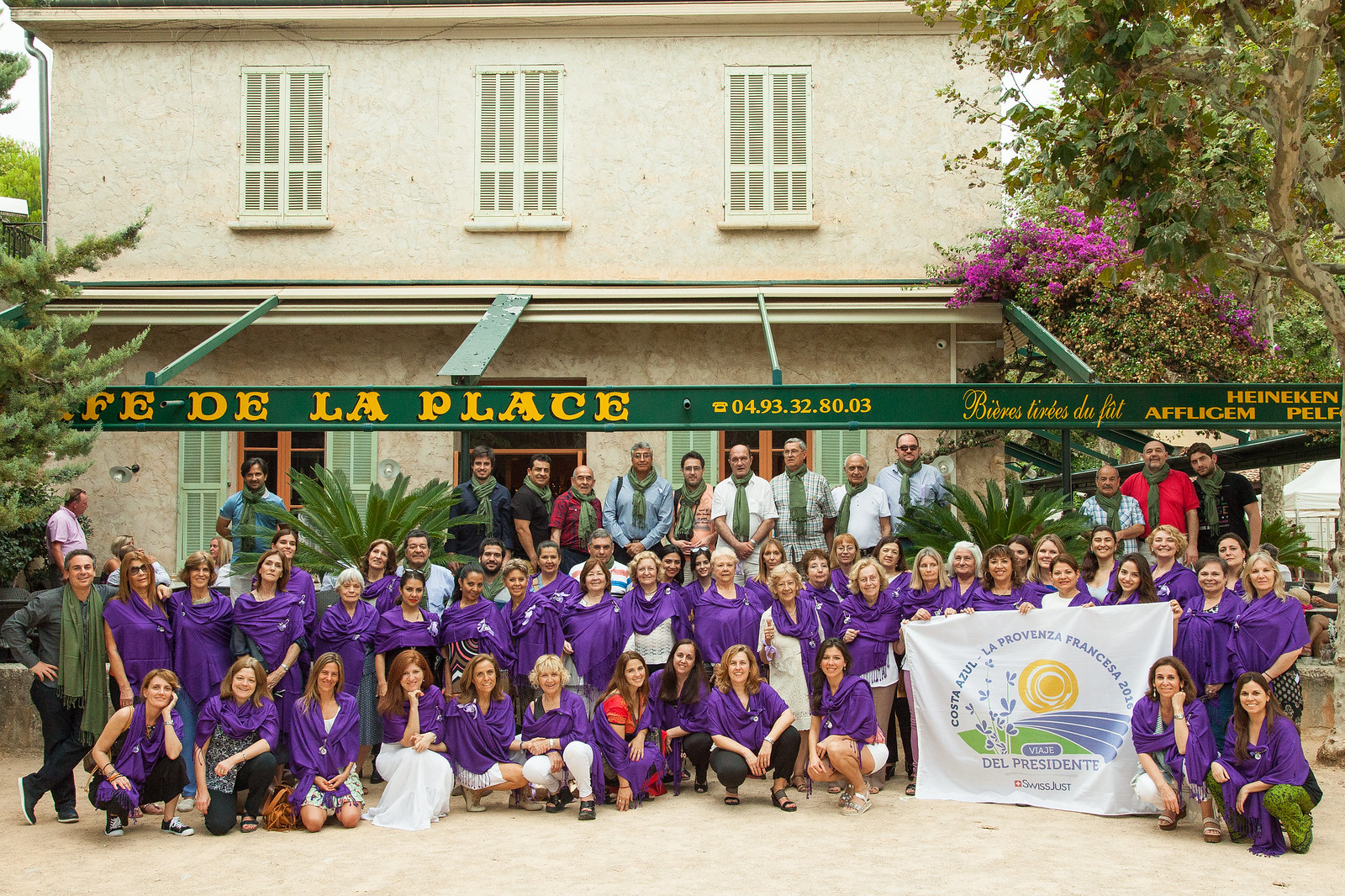The image captures a large group of approximately 40 to 50 people, predominantly women, posing outside a white building with a green awning inscribed with "Cafe De La Place" and a telephone number, 0493328003. The women, arranged in rows with the front row kneeling, are all dressed in purple garments resembling sashes, shawls, or tops. On the right side of the image, several women are holding up a white banner that reads "Costa Azul La Provenza Francesca 2016" with additional text "Del Presidente." The banner also features an animated sun and blue flowers. In the back rows stand several men, distinguishable by their green scarves and dress shirts, who appear to be of Indian descent. The background includes trees with bright purple flowers, adding a colorful touch to the daylight scene.